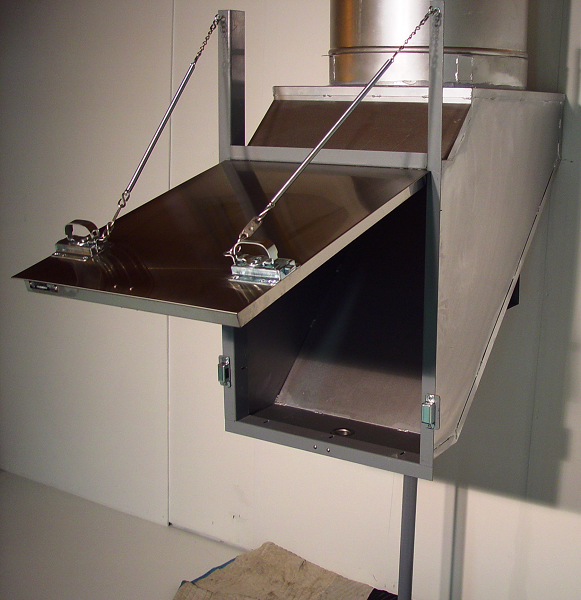This photograph showcases a commercial-grade metal chute system, possibly a trash or laundry chute, affixed to a pristine white wall. The primary structure, a gleaming chrome or shiny metal duct, ascends vertically and is prominently supported by two metal rods and a chain mechanism. A unique feature is the hatch at the bottom of the chute, which is trapezoidal in shape with a dark brown front, equipped with shiny metal handles. This hatch can be locked, thanks to the presence of locking mechanisms on either side. The arrangement suggests that the chain assists in holding the hatch open, counteracting gravity. The floor beneath the assembly appears bare, with a piece of wood or cardboard lying directly underneath the hatch, adding a practical element to the scene. The overall composition of the photograph is dominated by the sleek, industrial aesthetic of the chute's silver-grey metal and the starkness of the white background.